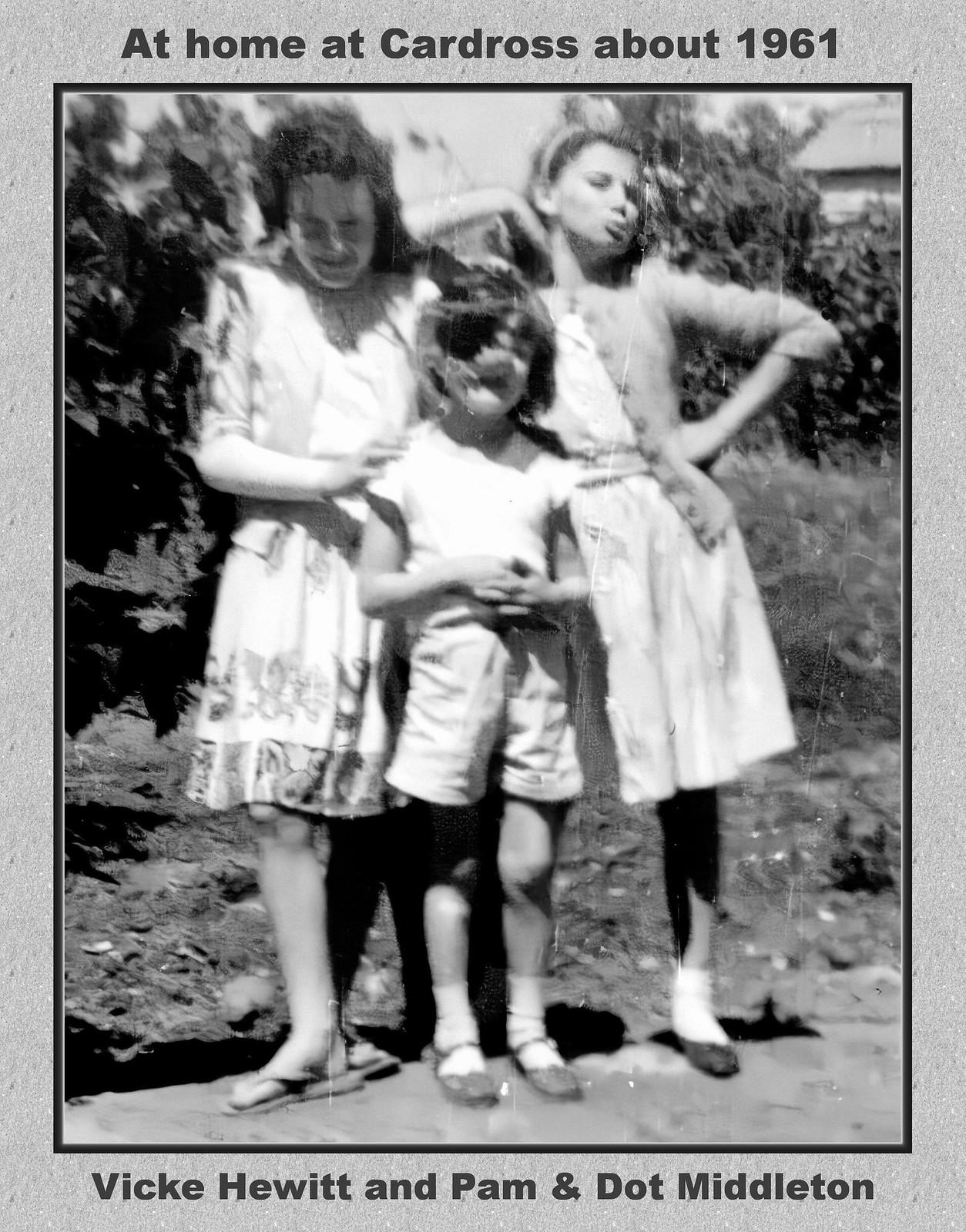This is an old black-and-white photograph presented on a textured light gray background resembling granite. The photograph is bordered by a thin black line with black text above and below it. At the top, it says "At home at Cardross, about 1961." Below the photograph, it reads "Vicki Hewitt and Pam and Dot Middleton."

The image features three females standing outdoors in front of trees, grass, and bushes. On the left is an adult woman with dark curly hair, wearing a floral dress and flip-flops. In the center is a young girl with dark short hair, dressed in a white shirt, shorts, white socks, and Mary Jane shoes. On the right is an older child or young woman, who might be blonde, wearing a long white dress with a sweater over it, white socks, and black flats. She is posing for the camera with her lips pursed and her hand up by her hair. The photo is somewhat blurry, adding to its nostalgic charm.